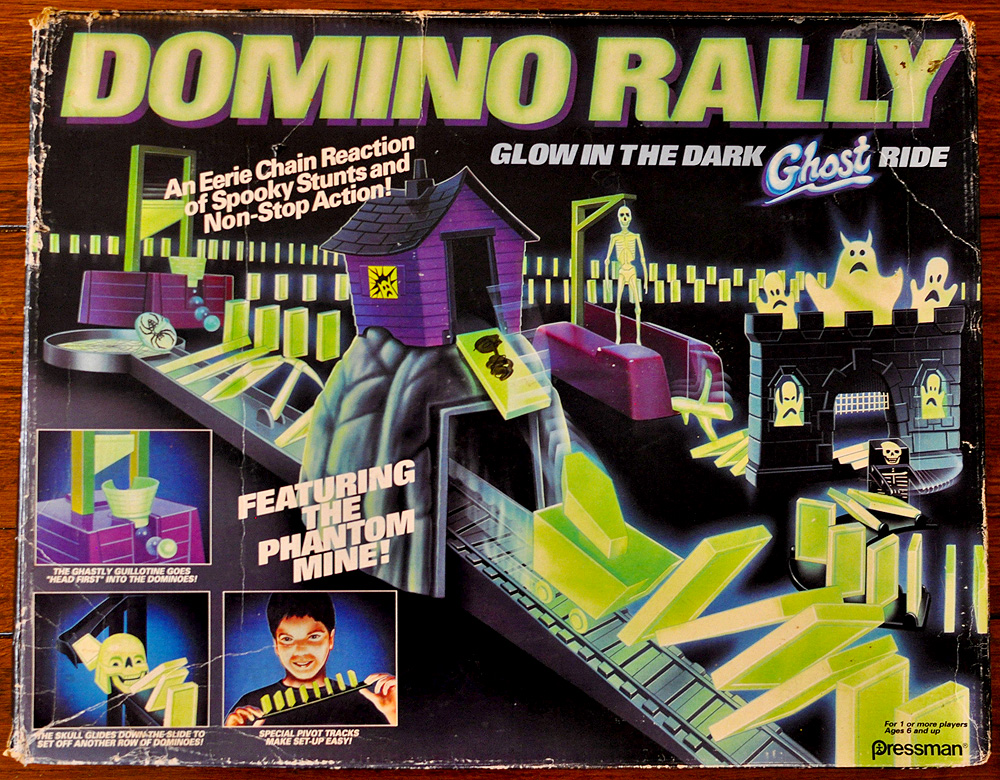The image showcases a vintage toy box cover for "Domino Rally: Glow-in-the-Dark Ghost Ride," featuring an eerie chain reaction of spooky stunts and non-stop action. The cover has a brown border and a black background. At the top, the title "Domino Rally" is displayed in yellow, with "glow-in-the-dark ghost ride" written beneath it. The left side has the tagline "An eerie chain reaction of spooky stunts and non-stop action" running diagonally. The bottom right corner is labeled with the brand name, Pressman.

The box art depicts a haunted Halloween theme with various spooky elements. A purple haunted house with a black roof stands prominently, surrounded by skeletons, ghosts, and lime green dominoes. These dominoes weave through different haunted setups, including an eerie castle with a drawbridge gate. There’s a grim cemetery with headstones made of dominoes, a glowing skull, and an interested young boy tipping dominoes on a slanted scale. The features also include a guillotine, a noose, and a trap door—all triggered by the dominoes. The phrase "Featuring the Phantom Mine" is displayed on the left side, enhancing the spooky and interactive experience of this vintage game box.